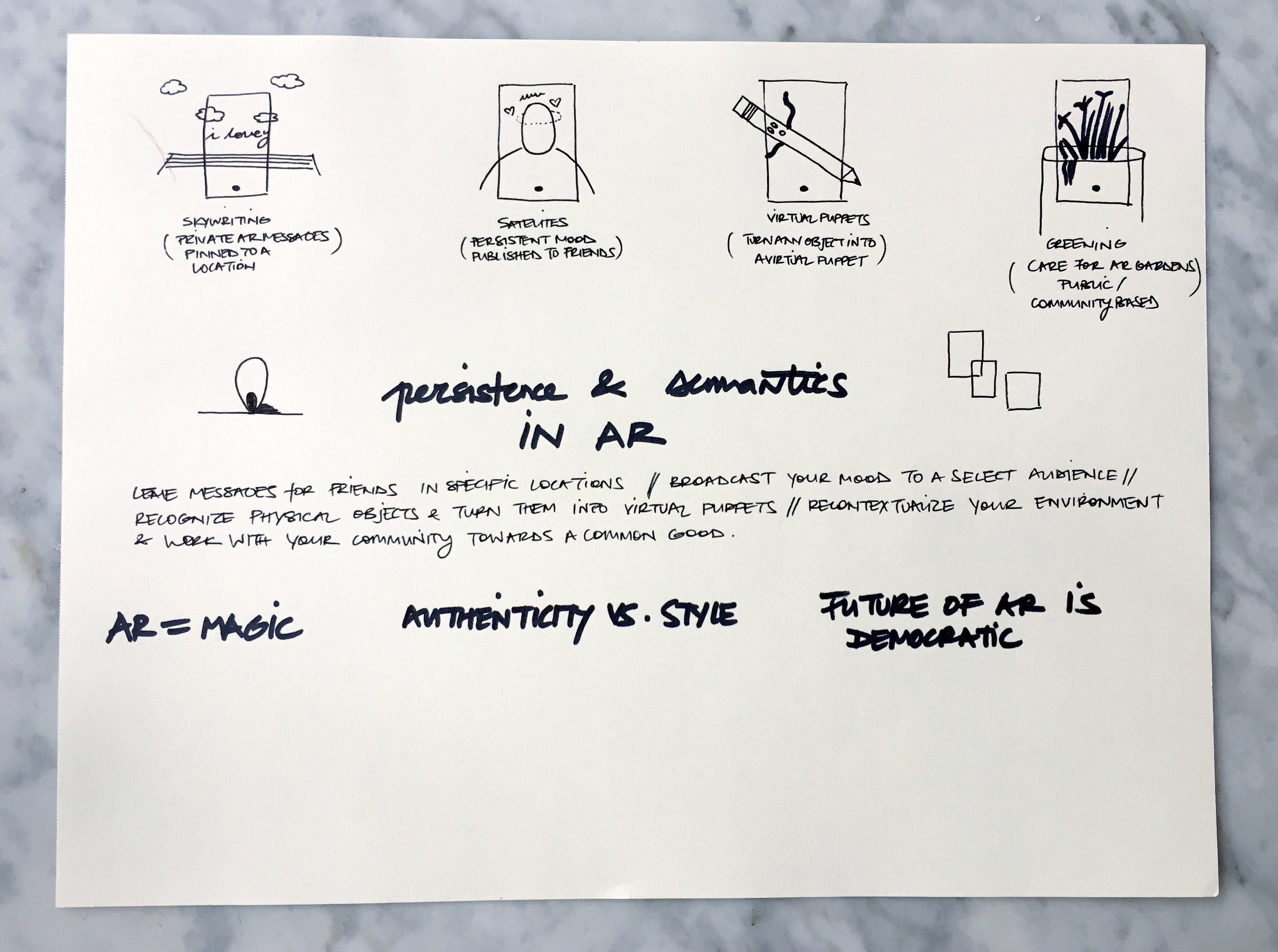This detailed caption focuses on the repeated elements and shared details from the sources:

This image is a horizontal color photograph of a white piece of paper, adorned with a series of drawings and written notes, resting on a marble surface. The paper contains a mix of illustrations and handwritten text in black pen and magic marker. In the upper left corner, it features the heading "Skywriting, private AR messages pinned to a location" alongside a sketch. From left to right across the top, the page includes several notable elements: a drawing labeled "Satellites, persistent mood, published to friends" next to an illustration of a person with hearts around their head, a pencil sketch accompanied by the words "Virtual puppets, turn an object into a virtual puppet," and a depiction of flowers with the caption "Greening, care for gardens, public community." 

Central to the paper is the prominent phrase "Persistence and semantics in AR," followed by more detailed descriptions and conceptual ideas about augmented reality (AR): "Leave messages for friends in specific locations, broadcast your mood to a secret select audience, recognize physical objects and turn them into virtual puppets, recontextualize your environment, and work with your community toward a common good." Additional key points highlighted include "AR equals magic, authenticity versus style," and "The future of AR is democratic." Collectively, these elements form an informative storyboard centered on the potential and aspirational aspects of AR technology.